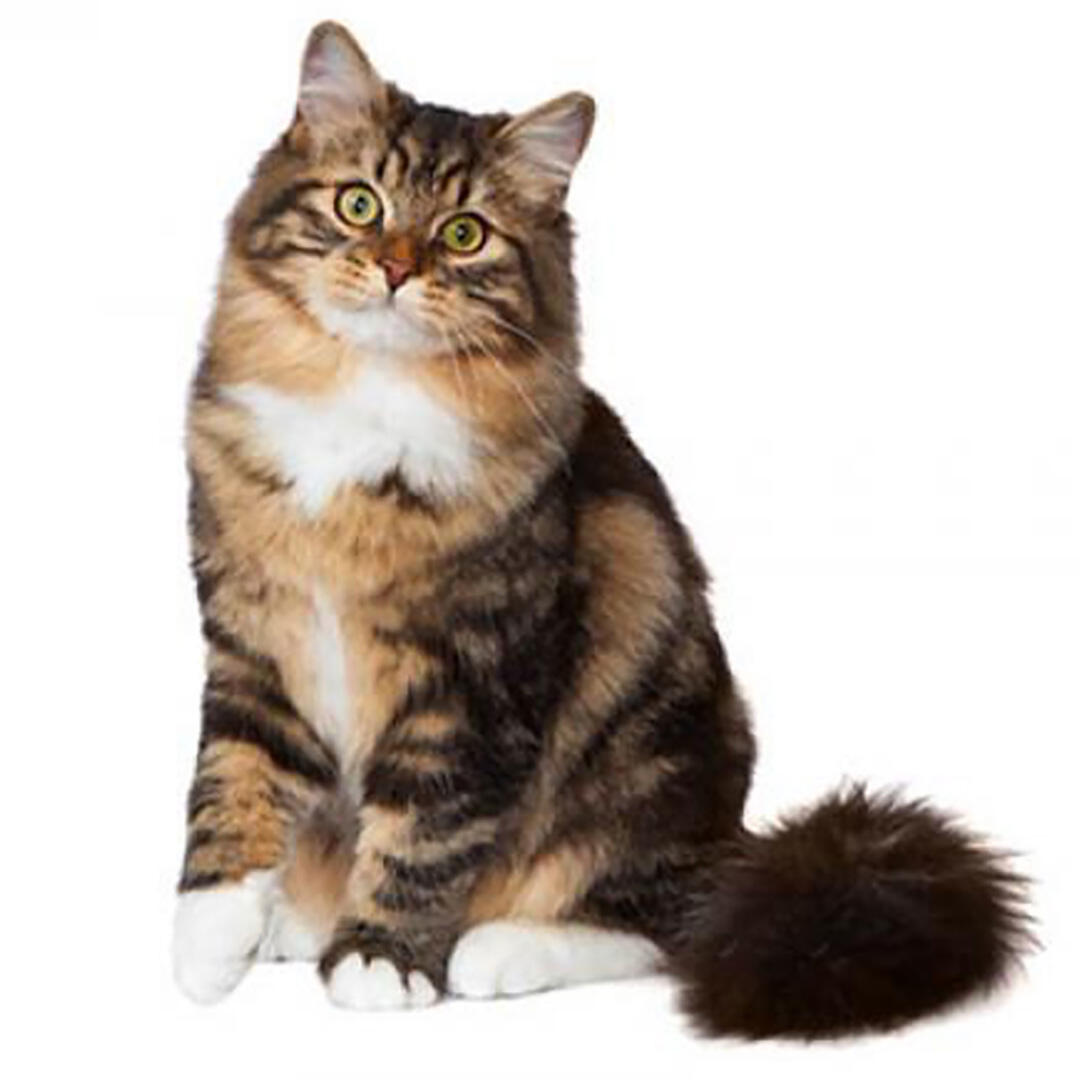This photograph features a single, multicolored calico cat seated on a white background. The cat, facing the camera with a slightly tilted head, showcases striking olive green eyes with yellow outlines, and ears perked up attentively. Its fur is a captivating blend of colors, with white paws, a predominantly dark brown head with light brown accents near the cheeks and nose, and an orange-pink nose. The cat's chest has an orangish-brown hue interrupted by a white blaze, while its body features a mix of dark and light brown stripes and spots, particularly on its right side that transitions from white to dark brown, tan, and various browns in a seemingly patterned sequence. The left leg mirrors this pattern but with brighter, almost orange, sections. All paws are white, with the front right paw lifted slightly off the ground, adding to its curious demeanor. The fluffy, dark brown tail curls around its body towards the bottom right of the image, accentuating the cat's regal and elegant posture.